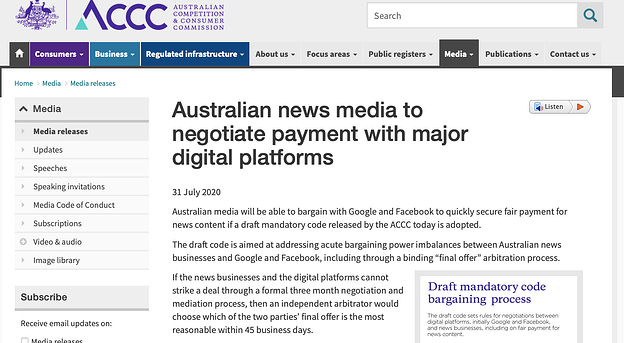The webpage appears to belong to the Australian Competition and Consumer Commission (ACCC). The theme of the page features a primarily white background with black text and accents of blue, purple, and green. At the top left, there is an icon or emblem resembling the letter 'A', followed by "CCC," indicating the ACCC. To the right, there is a prominent white search bar with a magnifying glass icon for searching the site.

Beneath the header, there are several navigation tabs including: "Consumers," "Business," "Regulated Infrastructure," "About Us," "Focus Areas," "Public Registers," "Media," "Publications," and "Contact Us." The "Media" tab is currently highlighted.

The main content of the page features a media release article titled "Australian News Media to Negotiate Payment with Major Digital Platforms," dated July 31, 2020. The article explains that Australian media organizations will soon be able to negotiate fair payment terms with Google and Facebook for their news content, contingent upon the adoption of a draft mandatory code released by the ACCC. The aim of the draft code is to address significant bargaining power disparities between Australian news businesses and major digital platforms like Google and Facebook. The proposed code includes a binding final offer arbitration process to resolve negotiations if the parties fail to agree within a formal three-month timeframe. Should negotiations and mediation fail, an independent arbitrator will select the most reasonable final offer between the two parties within 45 days.

On the left side of the page, the media section is elaborated with various options: "Media Releases" (highlighted), "Updates," "Speeches," "Speaking Invitations," "Media Code of Conduct," "Subscriptions," and "Video and Audio" links, alongside an "Image Library." Below this, there’s a subscription section where users can check a box to receive email updates.